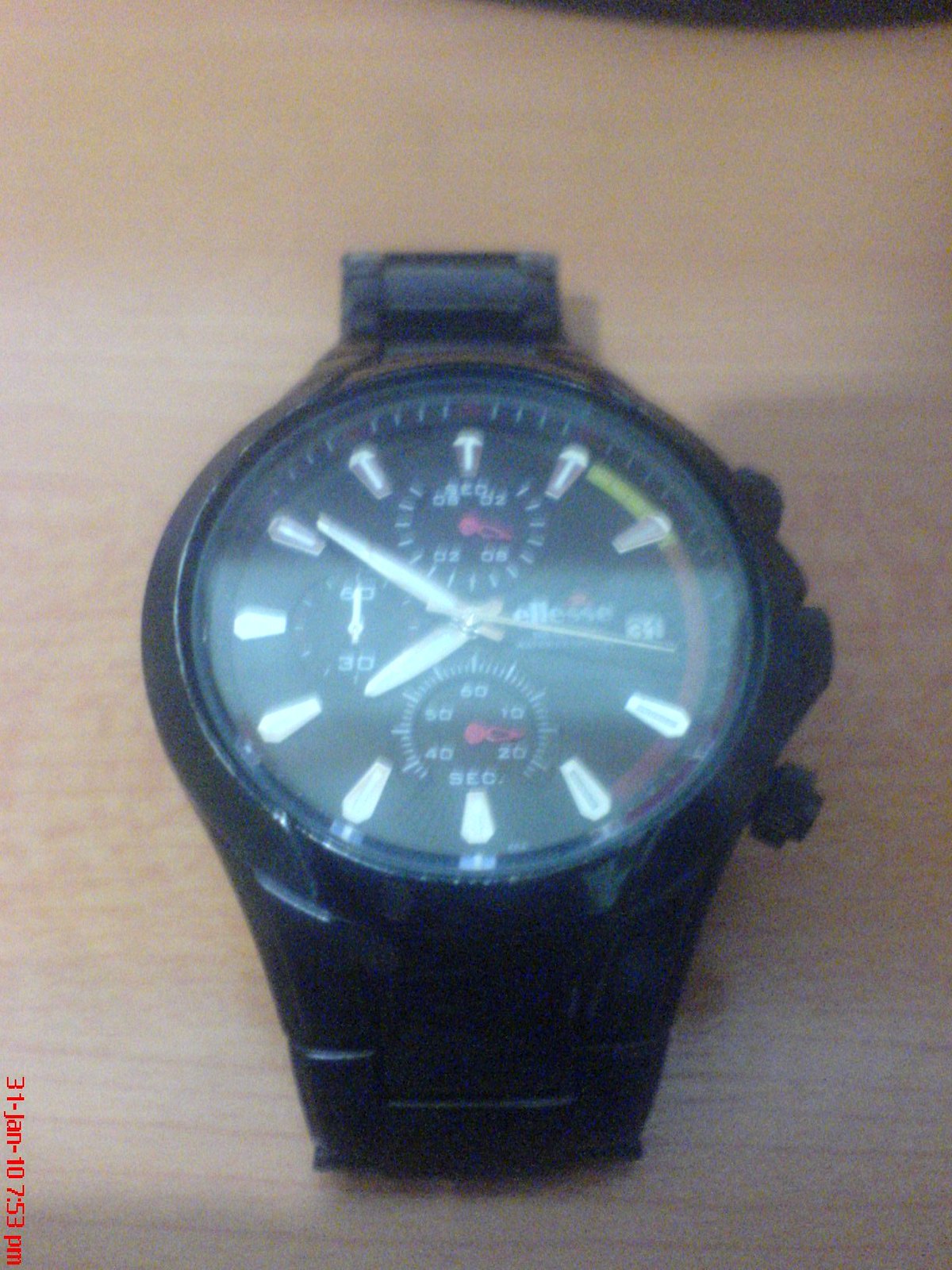This image is a photograph of an analog sports wristwatch with a black, ridged band, likely made from a stainless steel material. The watch's face is predominantly black, with a covering glass that shows a noticeable glare. It features three sub-dials inside: one marked with "60" and "30", another with "2" and "6", and a third labeled with seconds marked from "60" down to "10" in increments of ten. The hour, minute, and second hands are detailed in a silver color. Instead of traditional numbers, the watch bears silver-banded markers at each hour position.

To the right of the watch face, there are two distinct color bars: the top bar is yellow, and the bottom bar is red. Additionally, a small adjustment knob is positioned in the bottom right-hand corner of the watch face. The watch displays the date, "31", and there is an inscription on its band, "ELLESSE". 

This watch appears to be sitting on a wooden surface. The left-hand corner of the image indicates the date and time the photo was taken: "31st January, 10:53 p.m.", shown in red digital print.